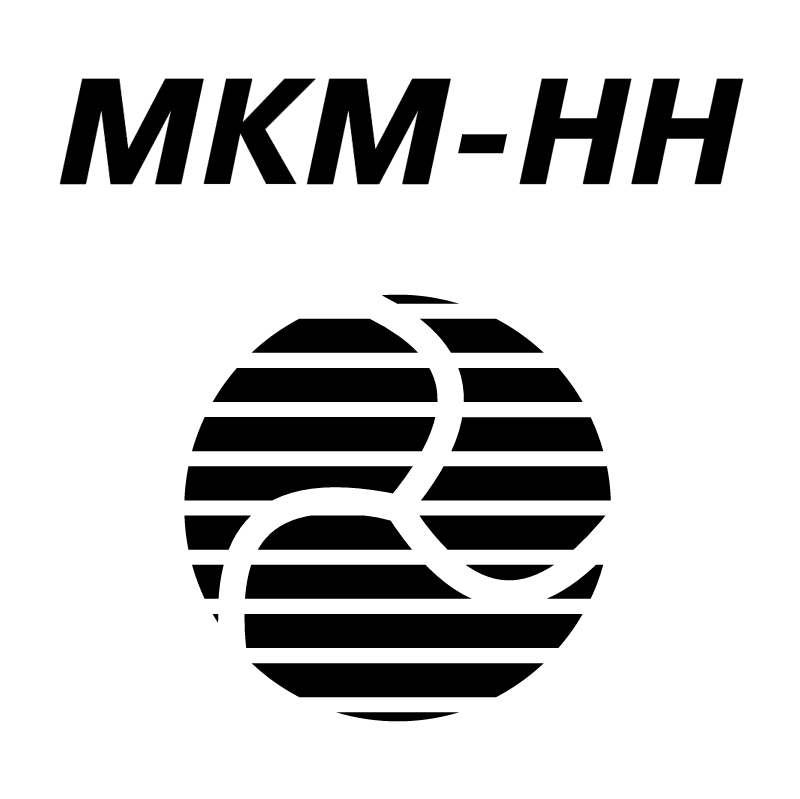The image showcases a company logo on a pure white background. At the top of the logo, the bold, black, capital letters "MKM-HH" are prominently displayed, slightly slanted to the right. Positioned centrally below the text is a distinctive circular design. This circular logo, composed of horizontally spaced black lines, portrays a disk with sections regularly cut out to create the pattern. Within this circle, intricate swirly lines extend from the center, forming three arm-like shapes that curve leftward. Additionally, smaller interconnected half-circles create an S-shaped pattern, further segmenting the interior of the main circle. The overall design suggests that it could be an emblem for a company or product line.